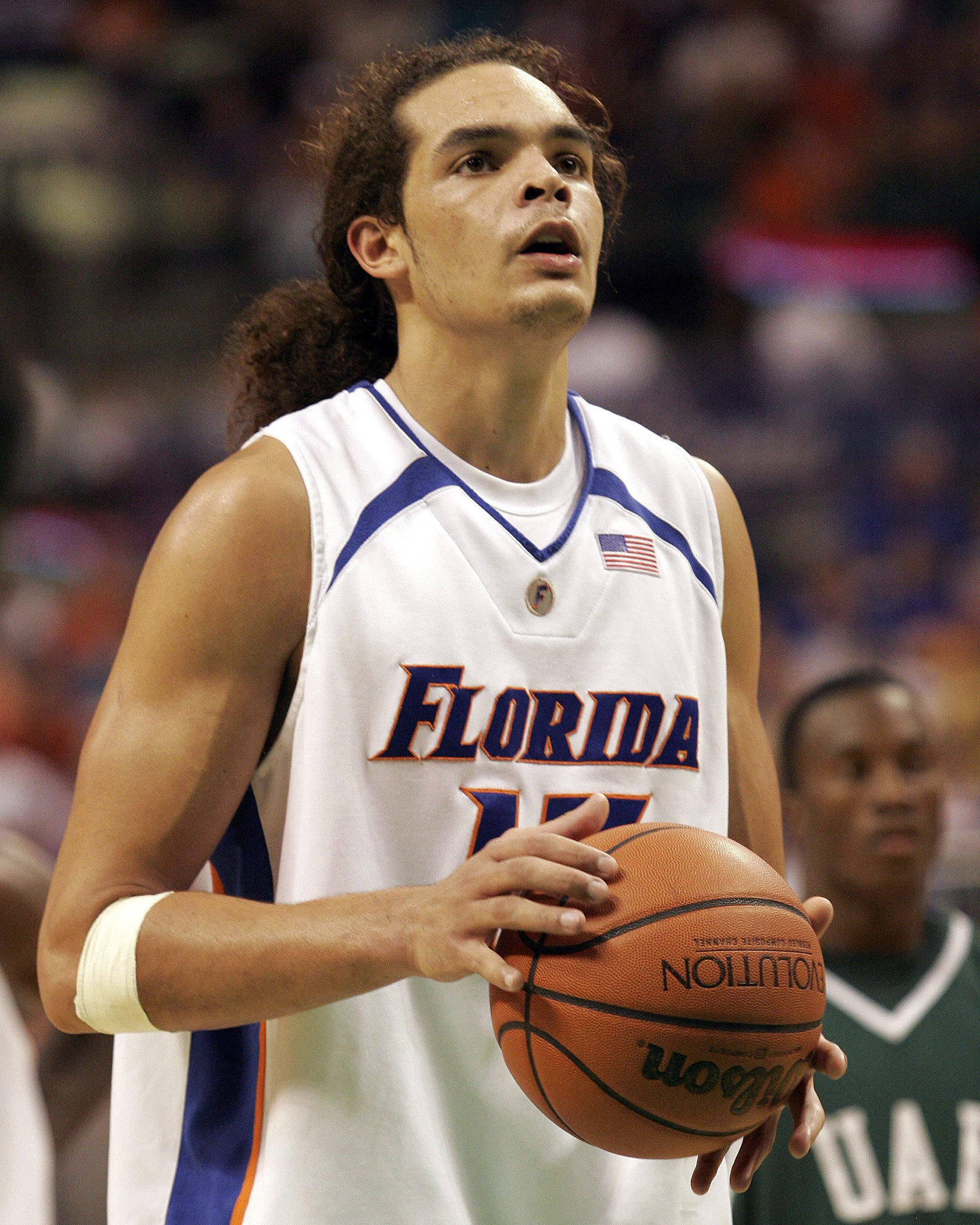The image captures a moment from an NCAA tournament game featuring a Florida University basketball player, who is preparing to take a free throw. The player, who is likely a young Joakim Noah, stands focused, holding a Wilson basketball in his hands. Dressed in a white, sleeveless jersey with "Florida" emblazoned in dark blue letters across the chest, he partially obscures the number beneath the text. His long brown hair is pulled back into a ponytail, and he wears a sports wrap below his right elbow. Visible on the left side of his chest are an American flag and a medallion with the letter "F." In the background, blurred spectators fill the arena, emphasizing the game's high-stakes nature as part of the March Madness tournament. To Noah’s right, a dark-skinned player from UAB, dressed in a green jersey with a white V-neck trim, watches intently.